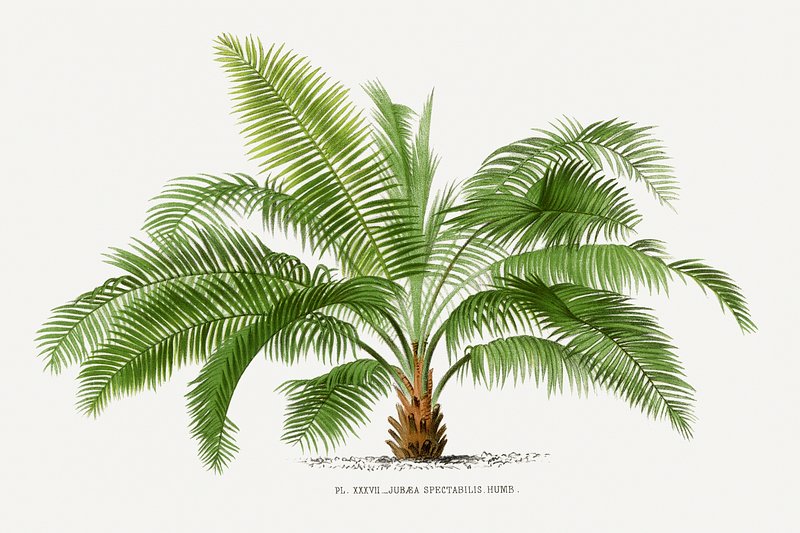This image is a digitally generated botanical illustration centered around a palm tree, Jubia spectabilis hum. The palm tree is depicted with a short brown base or stem, extending many green fronds in arched shapes prominently across the top and sides of the image. These fronds have a lush, green foliage reminiscent of those worn by hula dancers. The background is a light gray, almost white, and features a ground plane at the bottom indicated by dark brown speckles, possibly representing soil. There is small, gray typographic text at the base that reads "PL 37" and the scientific name "Jubia spectabilis hum." The overall style is consistent with botanical art, with a detailed, flat pattern in the foliage and a nature photography setting, despite the digital generation of the image.